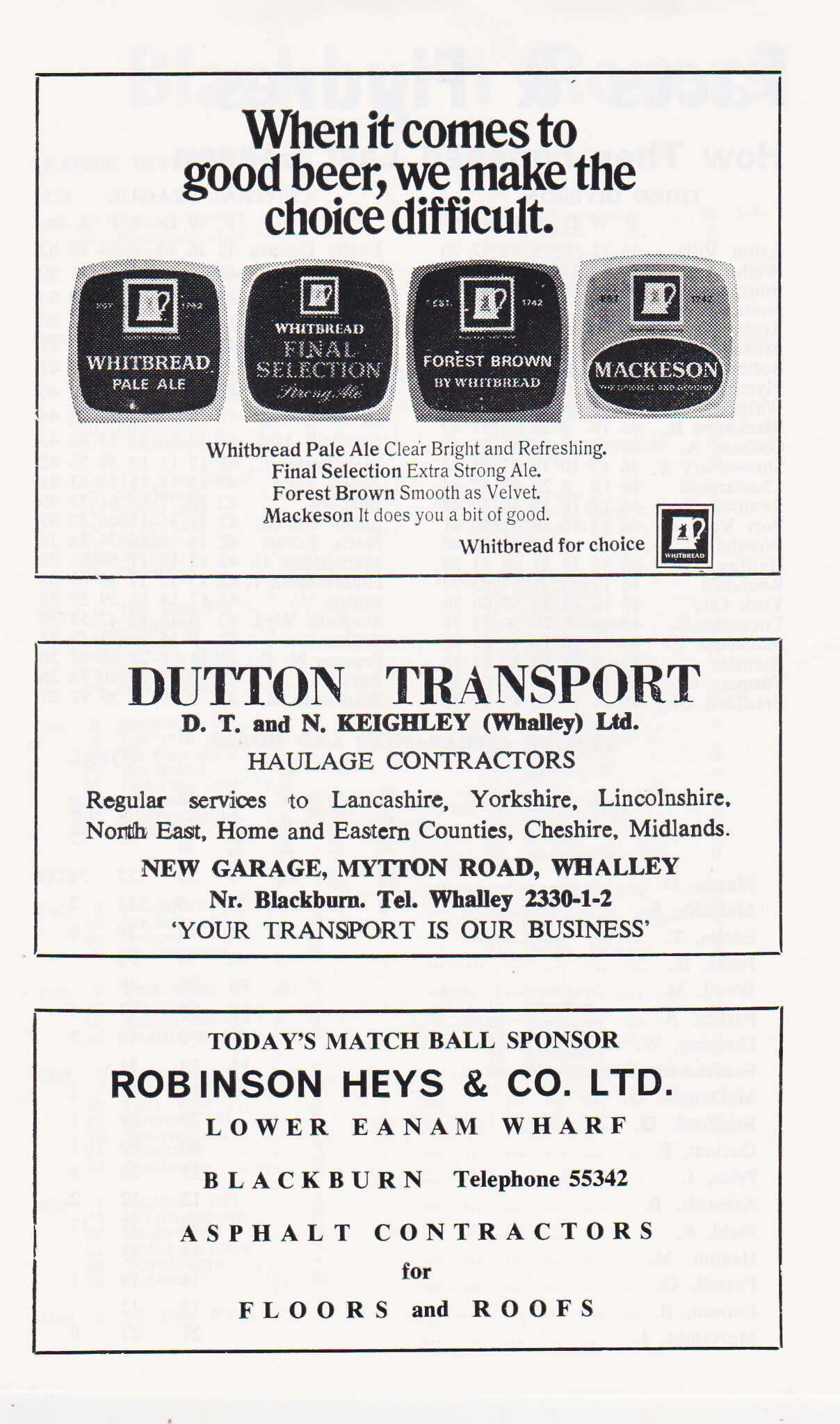The black-and-white image is an advertising page from a magazine or newspaper. Dominating the top portion of the page, black text reads, "When it comes to good beer, we make the choice difficult," followed by a list of beer labels: Whitbread Pale Ale, Final Selection, Forrest Brown by Whitbread, and Mackeson. Below these names, in smaller black text, additional descriptions are provided: "Whitbread Pale Ale, clear, bright, and refreshing. Final Selection, extra strong ale. Forrest Brown, smooth as velvet. Mackeson, it does you a bit of good. Whitbread for choice."

In a separate, distinct rectangle beneath, an ad for "Dutton Transport" includes the following details: "DT&N Keneally or Whaley Limited, Haulage Contractors, offering regular services to Lancashire, Yorkshire, Lincolnshire, Northeast, Home and Eastern Counties, Cheshire, and Midlands. New Garage, Mitten Road, Whaley, NR Blackburn. Telephone Whaley 233012. Your transport is our business."

Finally, at the bottom of the page, another advertisement announces: "Today's Matchball Sponsor is Robinson, Hayes & Co. Limited, Lower Enum Wharf, Blackburn. Telephone 55342. Asphalt Contractors for Floors and Roofs."